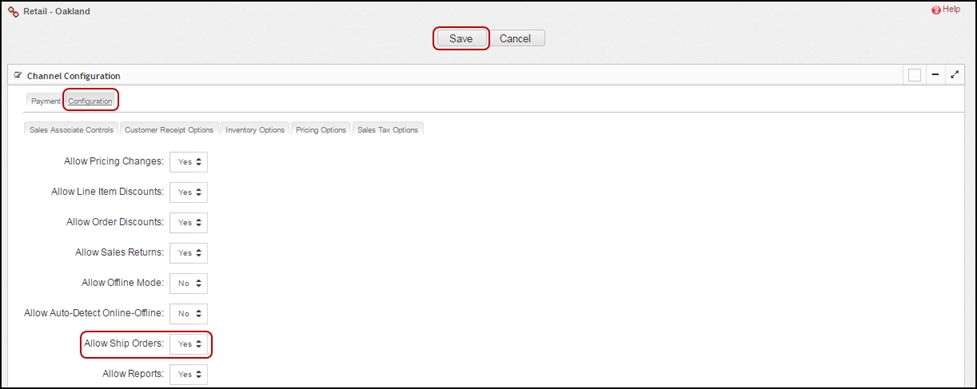This screenshot from a computer screen primarily features a gray background around the edges with a white central area filled with text in black and gray fonts. At the very top, the label "Retail-Oakland" is visible against the gray background. 

In the central white area, several interface elements are highlighted. A red rectangle outlines the "Save" button, while the adjacent "Cancel" button is not highlighted. Further down, the heading "Channel Configurations" is displayed prominently. Under this heading, the term "Payment-Con-Fountain" is partially circled with a red line, emphasizing the second word.

Towards the bottom of the screenshot, the phrase "Allow Ship Orders" appears, followed by an option set to "Yes." This section is also enclosed by a red rectangle for emphasis. The detailed red highlights and outlines serve to draw attention to specific interface elements and options within the software.